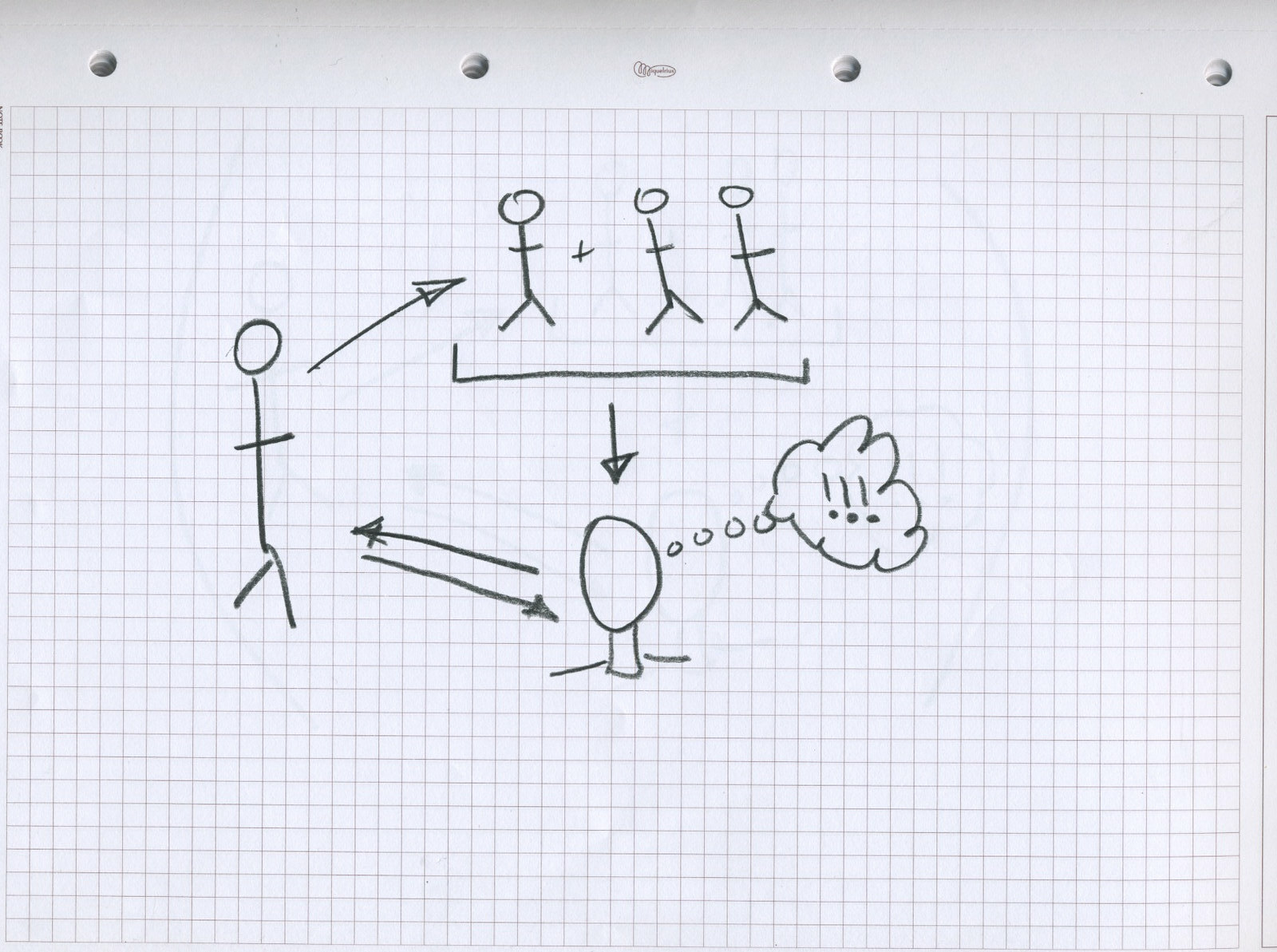This image depicts a sheet of graph paper oriented horizontally, with its four binder holes positioned at the top. Dominating the center of the graph paper is a marker-drawn illustration featuring a primary stick figure. An upward-right pointing arrow extends from this stick figure towards a smaller scene depicted above. This smaller scene consists of a smaller stick figure, a plus sign, and two additional stick figures, all enclosed by a bracket at the bottom. From this bracketed group, a black arrow points directly downward. 

Additionally, another black arrow runs horizontally from the main stick figure towards the right. Positioned below the clustered figures and to the right of the main stick figure, there is a head sketch without facial features, showing only the neck and partial shoulders. An arrow extends from this head back to the left towards the original stick figure. Intriguingly, the figure on the left is illustrated with small round circles and a cloud containing three exclamation marks, indicating an emotive reaction or thought.